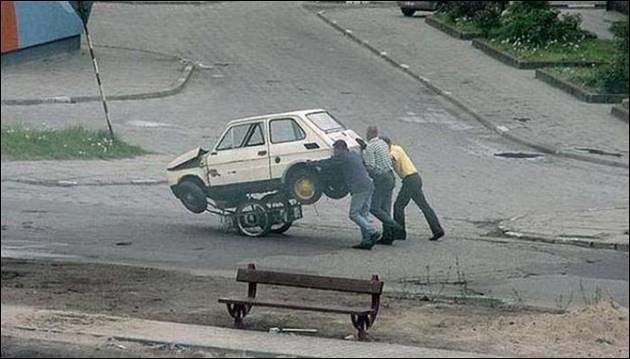This photograph captures a poignant scene in what appears to be a less affluent country. The setting is outdoors, dominated by a wide and somewhat neglected Y-shaped road with broad pavements and a gray brick sidewalk adorned with low, square planters filled with greenery, bushes, and a few flowers. The focal point is an antiquated, tiny car, likely a defunct Fiat or a similar model, in a dirty white or beige color. The vehicle has clearly been involved in an accident; its bonnet is badly damaged and protruding towards the windshield, with the front passenger side wheel nearly detached. Ingeniously, the car has been elevated onto a rudimentary metal frame with two wheels, resembling pram or bicycle wheels, to facilitate its movement. Three light-skinned men—one in a blue shirt and jeans, another in a white checked shirt and dark pants, and the third in yellow and black pants—are pushing the car from behind, navigating it sideways across the road. An empty bench sits in front of them as they struggle to maneuver the broken-down vehicle, highlighting a scene where traditional roadside assistance appears absent.